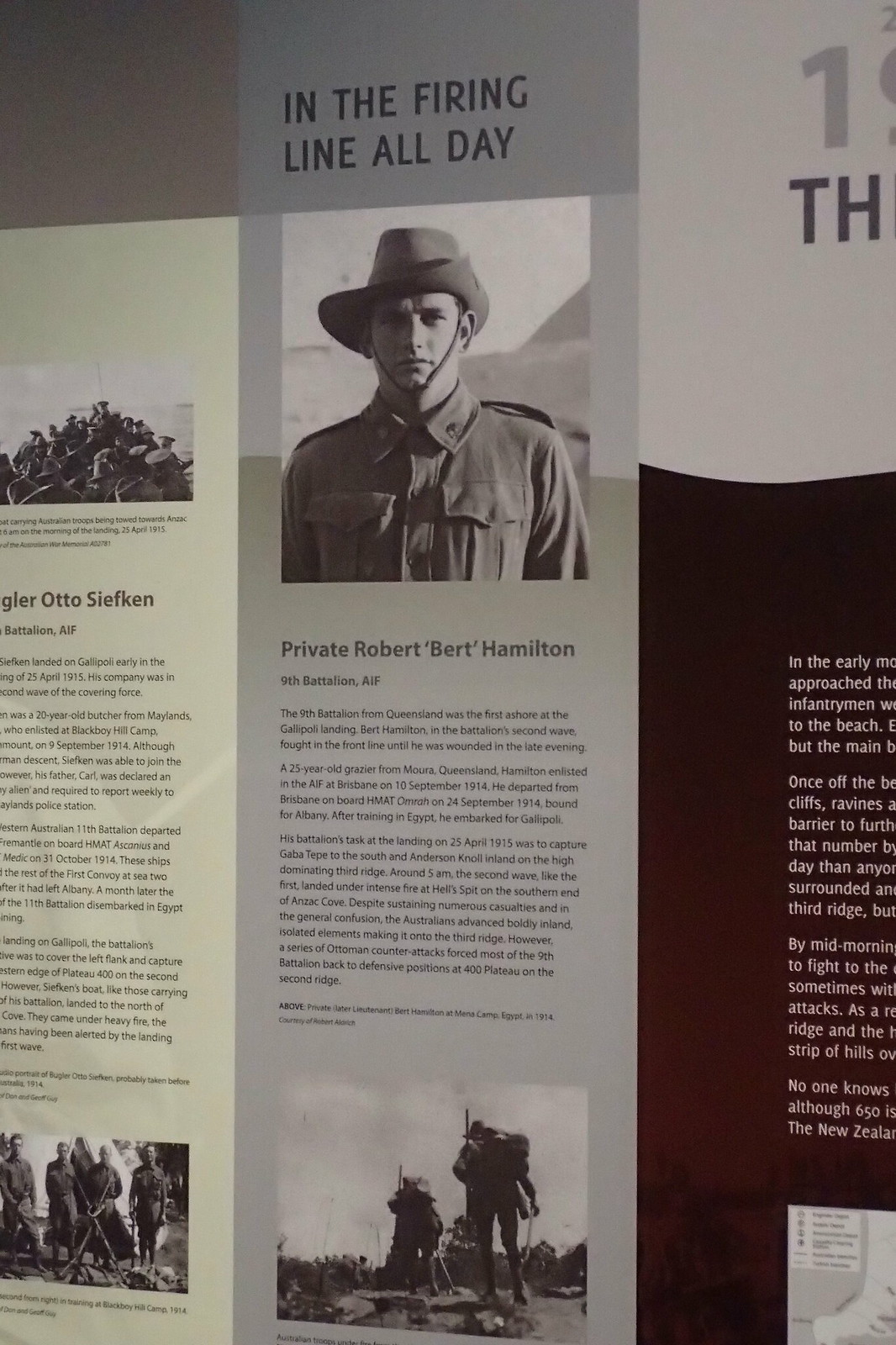In this black and white photograph, situated in the upper middle portion of the image, is a man wearing a cowboy hat. Above him, the words "In the Firing Line All Day" are prominently displayed. This man, identified as Private Robert Burt Hamilton from the 9th Battalion, AIF, appears to be the central figure. Underneath his image, the caption reads, "Private Robert Burt Hamilton, 9th Battalion, AIF." Hamilton, a 25-year-old glazer from Mora, Queensland, was part of the Battalion's second wave during the Gallipoli landing and fought in the front line until he was wounded in the late evening. The image is accompanied by an article about him, with additional articles about others positioned to the left and right of his image, all suggesting that this collection of narratives is part of a magazine spread. The left side shows a picture of a group of men, further contextualizing the historical significance of the scene.